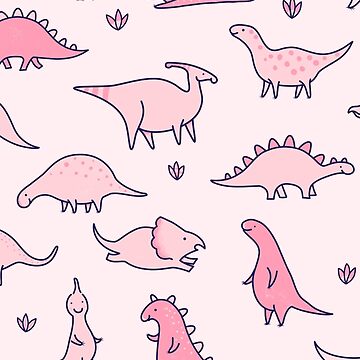This image is a vibrant and playful cartoon rendering of various dinosaur species, designed as a pattern that could adorn a child's bedroom as wallpaper or decorative paper. The background is a very light beige in some interpretations and shades ranging from light pink to medium and dark pink in others, providing a soft and inviting backdrop. The dinosaurs are depicted in different shades of pink and purple, including identifiable species such as stegosaurs, hadrosaurs, tyrannosaurus rex, triceratops, and other fictional or imaginative dinosaurs. Some dinosaurs feature distinctive characteristics like little horns and spikes running from their heads down to their tails. Interspersed among the dinosaurs are charming little graphics of plants and three-leafed patterns, enhancing the overall playful aesthetic. The images are arranged in a non-repeating, random pattern, which adds to the whimsical and youthful feel of the design. The style appears childlike, either drawn by children or crafted by an artist aiming to mimic a child's drawing style, making it visually engaging for young viewers.